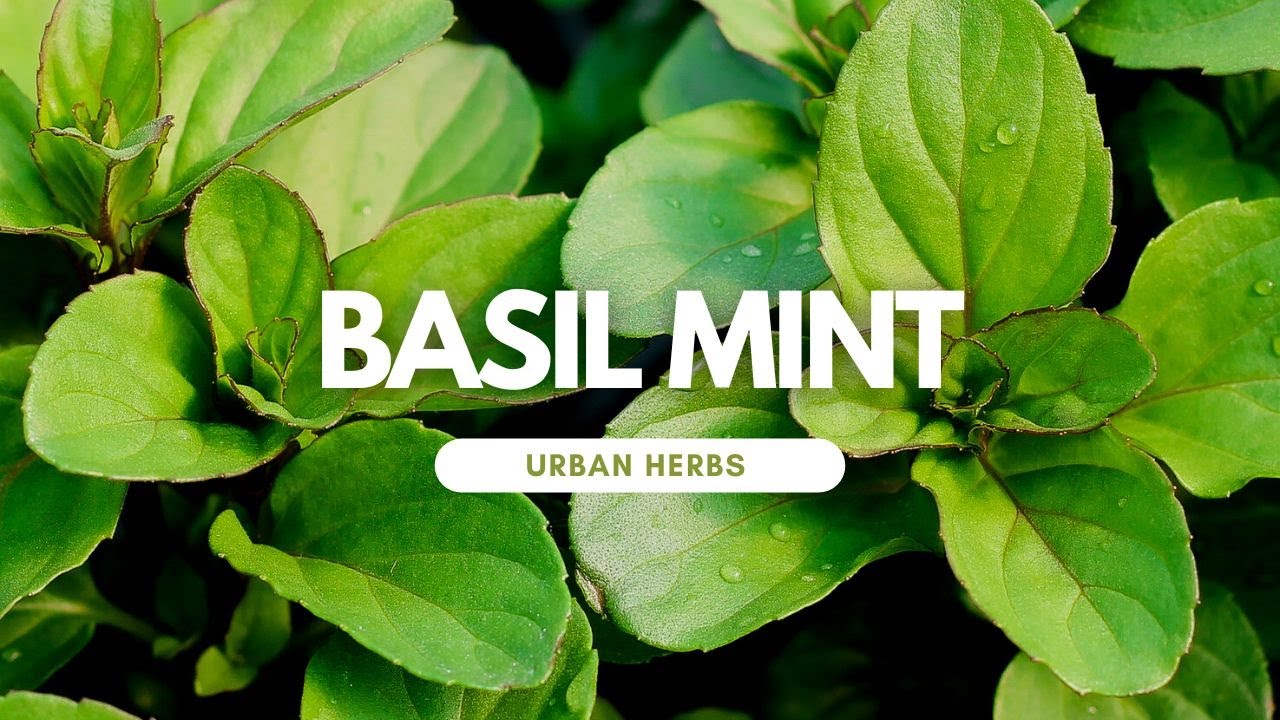The image features an advertisement for Basil Mint, prominently showcasing lush, vibrant mint plants against a dark background. The leaves are a mix of jade green and light green shades, some with white edges and centers. Water droplets are visible on the leaves, suggesting they have just been watered or are kept in a humid environment. Dominating the center of the image, bold white text reads "Basil Mint." Below this, a white pill-shaped blur houses the green capital letters spelling "Urban Herbs." The overall impression is a serene, focused view on the fresh, dewy mint leaves with no other elements in the backdrop.